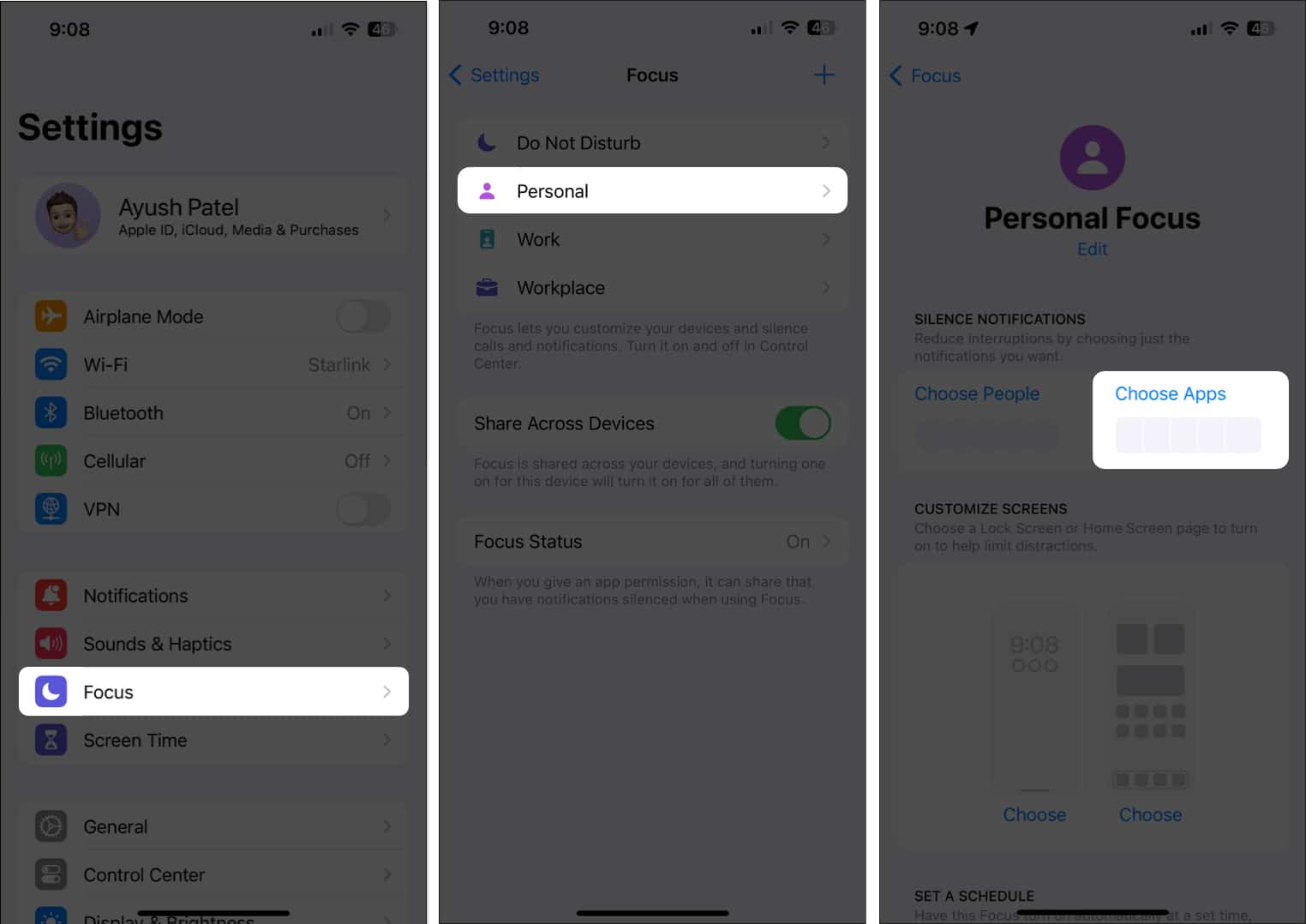This triptych illustrates a detailed walkthrough of mobile application settings across three stages. 

From left to right:
1. **First Screenshot**: Depicts the general settings page with a user icon for Ayush Patel, labeled with options for Apple ID, iCloud, Media, and Purchases. The settings are categorized with colorful icons as follows:
   - Airplane Mode
   - Wi-Fi
   - Bluetooth
   - Cellular
   - VPN
   - Notifications
   - Sounds and Haptics
   - Focus (Highlighted)
   - Screen Time
   - General (partially cut-off)
   - Control Center (partially cut-off)

2. **Second Screenshot**: Focuses on the 'Focus' settings. Displaying another set of categories, each with distinctive icons:
   - Do Not Disturb
   - Personal (Highlighted)
   - Work
   - Workplace
   The 'Personal' section is highlighted, featuring a white background, a purple person icon, and an arrow pointing to the right.

3. **Third Screenshot**: Delves deeper into the 'Personal Focus'. The page title reads 'Personal Focus', with an 'Edit' option in blue text beneath. The highlighted section is a blue 'Choose Apps' link located centrally on the right part of the screen, followed by five gray rectangles meant for app selection, with the two outermost rectangles having rounded corners.

This progression effectively guides the viewer through the steps from the main settings to selecting specific focus modes, culminating in the customization options available within the 'Personal Focus' settings.